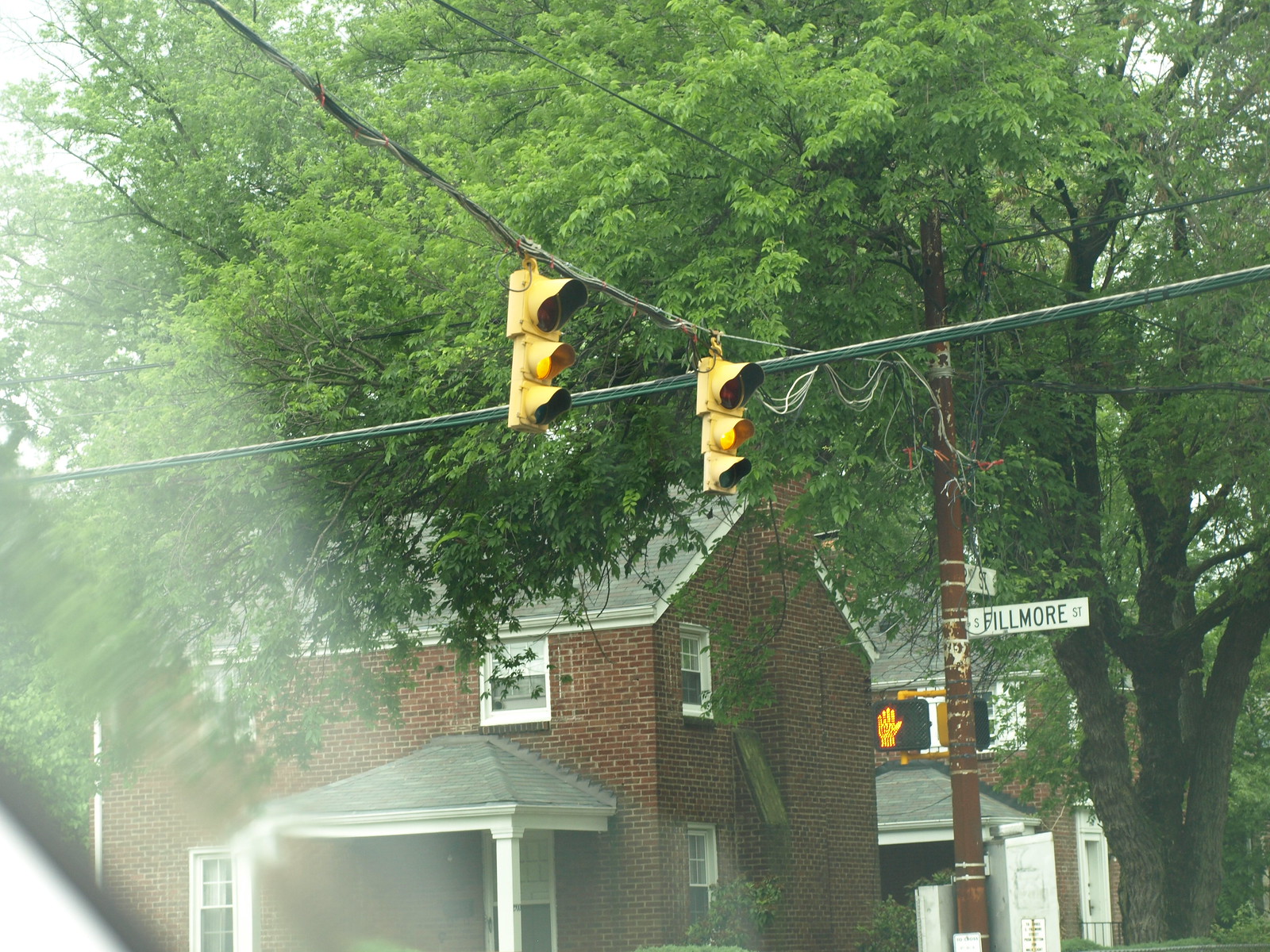In this rectangular daytime photograph, we see a charming urban scene featuring several red brick buildings that appear to be either apartments or single-family homes. The architectural style suggests these structures were built in the early 1970s. Prominently in the lower left foreground, a two-story home showcases white painted windows and trim, complemented by an overhang sheltering the front door. Another building of similar style is partially visible in the background.

A double streetlight, suspended horizontally by wires, stretches across the scene, with additional wires running both vertically and horizontally throughout the image. On the right corner of the home, there is a dark red street post or telephone pole. Affixed to this post is a white street sign with black text, indicating Fillmore Street running east to west. Below this, another sign partially reads "ST", though the full name is obscured.

The upper half of the image is dominated by lush greenery from mature trees, likely elms, their fully-leaved branches providing a rich canopy. These trees add a verdant contrast to the urban brickwork, creating a harmonious balance between natural and built environments.